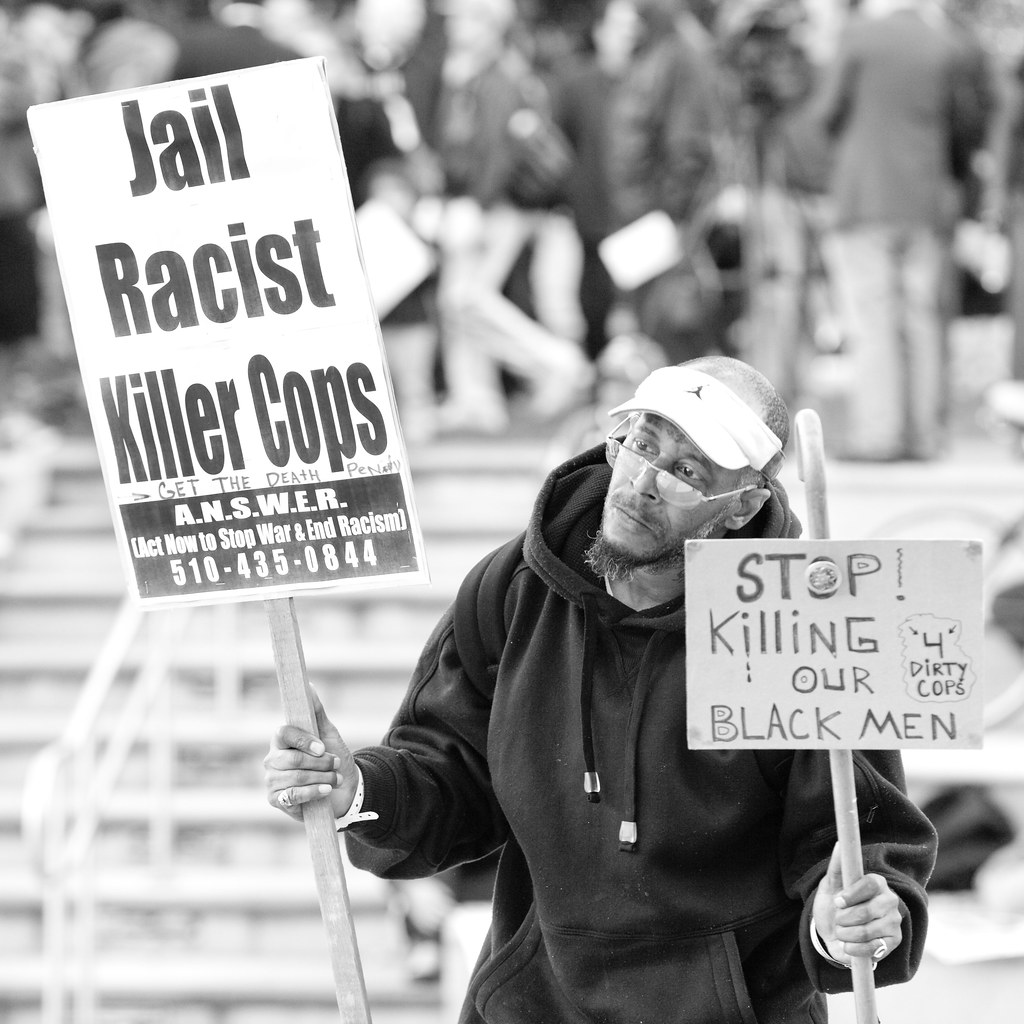In this black and white photograph, an older, balding African American man is depicted standing outdoors, likely during a protest in the middle of the day. He is wearing a black sweatshirt with drawstrings and a white visor featuring a black icon in the center. The man is central to the composition, holding two distinct signs. The left sign reads, "Jail Racist Killer Cops. Get the Death Penalty. A.N.S.W.E.R. Act Now to Stop War and End Racism," along with the phone number 510-435-0844. This message appears to be professionally printed. The right sign, which seems to be handmade and attached to a stick, declares, "Stop Killing Our Black Men for Dirty Cops." The background of the photograph is blurred but reveals a staircase with handrails, emphasizing the depth of field. The detailed protest signs and the stark, monochromatic tones contribute to the photograph's potent and urgent message against racial injustice and police brutality.